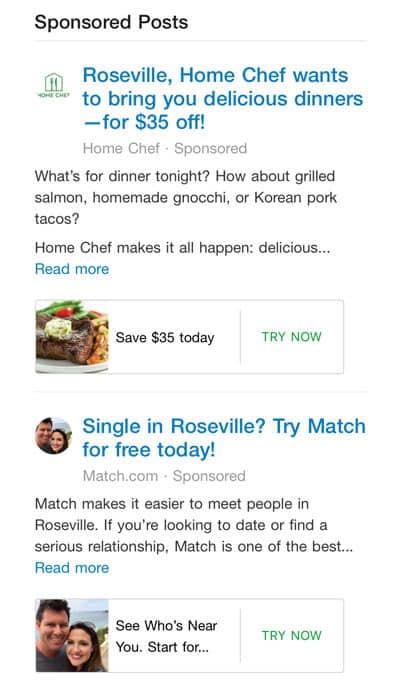This image is a sponsored post from the company Home Chef. At the top, the text "Sponsored Posts" appears in black, accompanied by the Home Chef icon and a blue heading stating, “Roseville, Home Chef wants to bring you delicious dinners for $35 off.” The post includes tempting meal suggestions such as grilled salmon, homemade ganache, and Korean pork tacos, with a call to action, "Home Chef makes it all happen. Delicious..." accompanied by a clickable "Read More" link.

Below the Home Chef promotional content is an image of a mouth-watering dish alongside the words "Save $35 Today" and a prominent "Try Now" button.

Further down, another sponsored ad appears from Match.com, targeting singles in Roseville. The ad claims, "Single in Roseville? Try Match for free today. Match.com Sponsored. Match makes it easier to meet people in Roseville. If you're looking to date or find a serious relationship, Match is one of the best..." with a "Read More" link provided.

At the bottom of the page, a Match.com photo features a smiling male and female, followed by the text "See Who's Near You, Start For..." and another "Try Now" button. For additional information, the ad directs visitors to match.com.